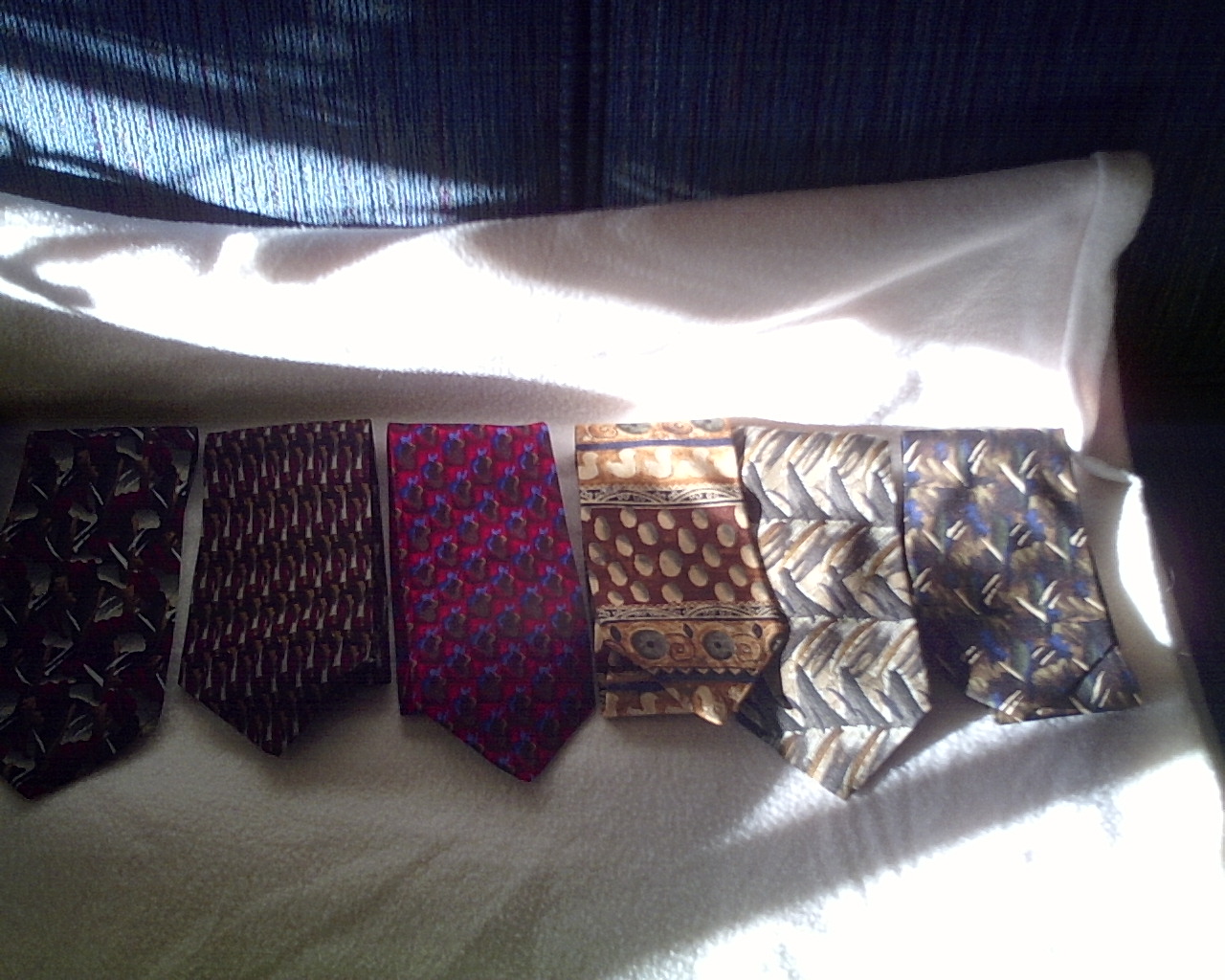The image showcases six neatly folded neckties, each displaying its unique design and color pattern. The ties are arranged on a white cloth placed on a blue couch or chair. There's light streaming in from a window, illuminating two of the ties while the others remain in shadow. The ties vary in color and material, potentially silk or polyester, with the following specific descriptions: 

- The first tie is a dark brownish color with complex, textured designs.
- The second tie features a black and tan pattern.
- The third tie boasts a combination of red, green, and white hues.
- The fourth tie is red and blue with floral patterns.
- The fifth tie is brown and gray, with some ties depicting ostrich feather-like patterns and another with ducks and white pebbles.
- The sixth tie combines black, brown, and blue colors.

The blue couch or chair against the equally blue wallpaper in the background creates a subtle, monochromatic setting for the vibrant and varied ties.